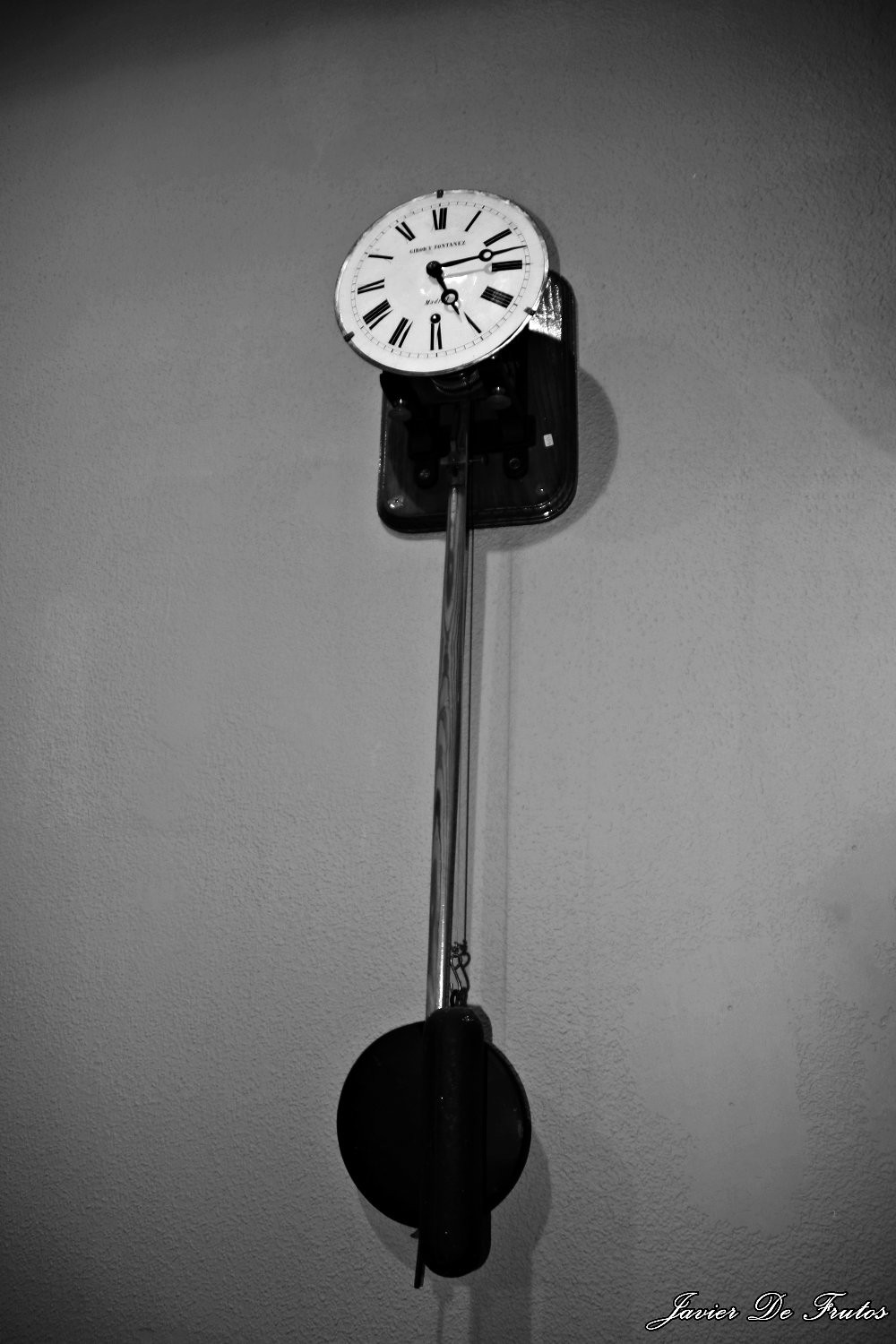This black-and-white photograph captures a unique and very old clock mounted on a wall with a lightly textured, gray background similar to flattened-out knockdown popcorn ceilings. The clock features a black rectangular base with a white clock face displaying black Roman numerals and two black hands, indicating the time as approximately 12 minutes past 5. The clock's exterior is framed in silver with clips securing the clock face. Below the black box, a long silver pendulum hangs, ending in a weight, reminiscent of a grandfather clock but without the wooden cabinet. Notably, the bottom right-hand corner of the photograph includes the name "Javier de Frutos" in elegant white cursive. Shadows cast to the right suggest lighting from the left, adding depth to the image.